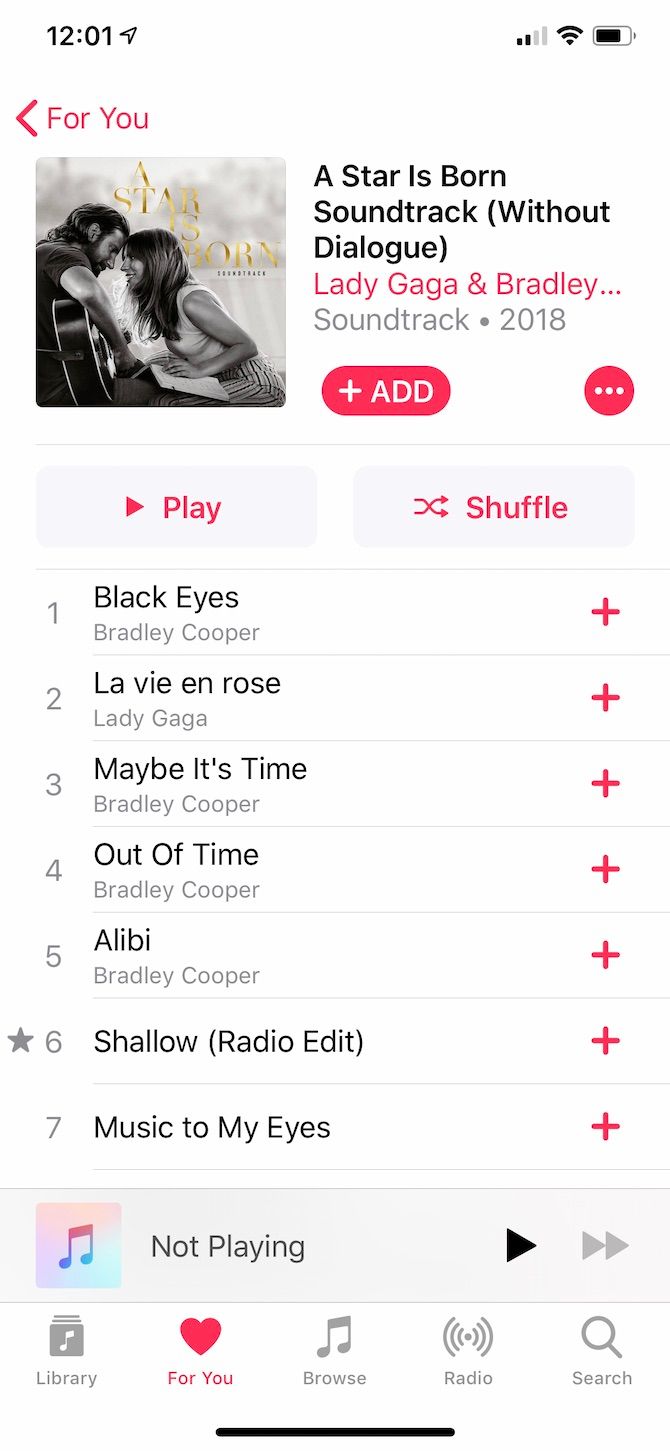In the upper left corner, the time is displayed as 12:01. In the upper right corner, there is a battery symbol that is almost completely filled with black color. To the left of this symbol, a small red arrow points left with the word "For You" in red text beside it.

The main portion of the image is a black-and-white still from the movie "A Star is Born," featuring Bradley Cooper holding a guitar and Lady Gaga leaning forward, their heads touching intimately. Below this image, in black text, it reads: "A Star is Born Soundtrack" with "2018, Lady Gaga and Bradley Cooper" in parentheses.

A red button invites interaction with "Click to Add" text. Beneath this, a list of songs from the soundtrack is displayed:
1. "Black Eyes" – Bradley Cooper
2. "La Vie en Rose" – Lady Gaga
3. "Maybe It's Time" – Bradley Cooper
4. "Out of Time" – Bradley Cooper
5. "Alibi" – Bradley Cooper
6. "Shallow (Radio Edit)" – marked with a star
7. "Music to My Eyes"

A small "plus" sign appears beside the track "Music to My Eyes," indicating an option to add the song. Adjacent to this is a music symbol inside a square with peach, purple, and blue colors. 

At the bottom, there is a black arrow highlighted beneath a red heart, with the text "For You" under it.